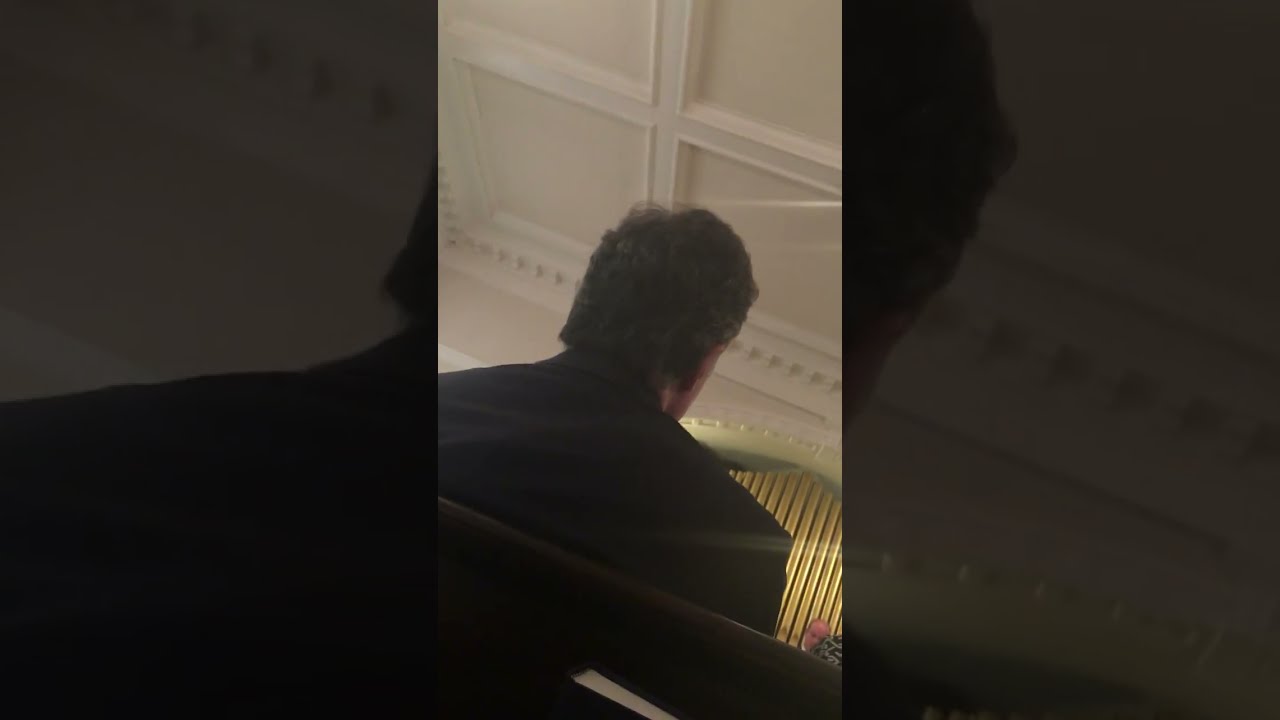The image depicts a cell phone photograph taken inside a church during a service. The setting is indoors, marked by a high-ceilinged space likely featuring an altar or stage area that is partially obscured in the background. In the foreground, the top of a wooden pew appears, complete with a holder containing two books, possibly hymnals or Bibles. Seated directly in front of the photographer, a man on the left in a dark jacket and a woman on the right in a black and gray print top obscure most of the view of the altar. 

The sermon is being delivered by a preacher whose head and shoulders are faintly visible between the two seated individuals. Behind the preacher, gold-colored organ pipes rise toward the ceiling, contrasting against the white background of the upper walls. The photograph is somewhat blurry and slightly tilted clockwise, adding to its unprofessional appearance. The scene is characterized by a mix of colors including gold, black, gray, white, brown, and beige.